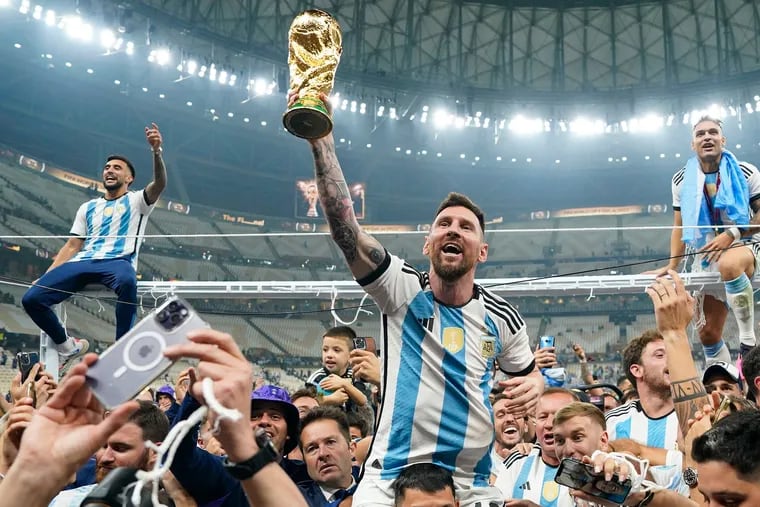The image captures the exhilarating moment of a soccer victory in an illuminated, mostly empty stadium. At the center, a man with a tattooed right arm - possibly Lionel Messi - is triumphantly holding up a golden trophy, likely the FIFA World Cup, while being elevated on a teammate's shoulders. He is proudly wearing a short-sleeved, blue and white striped Argentinian jersey. Surrounding him, a sea of people can be seen cheering, capturing selfies, and raising their phones to immortalize the moment. Two other players, also in the characteristic blue-striped jerseys, stand elevated on platforms above him. This scene vividly portrays a triumphant celebration, with the stadium lights casting a glow over the jubilant athletes and their fans.